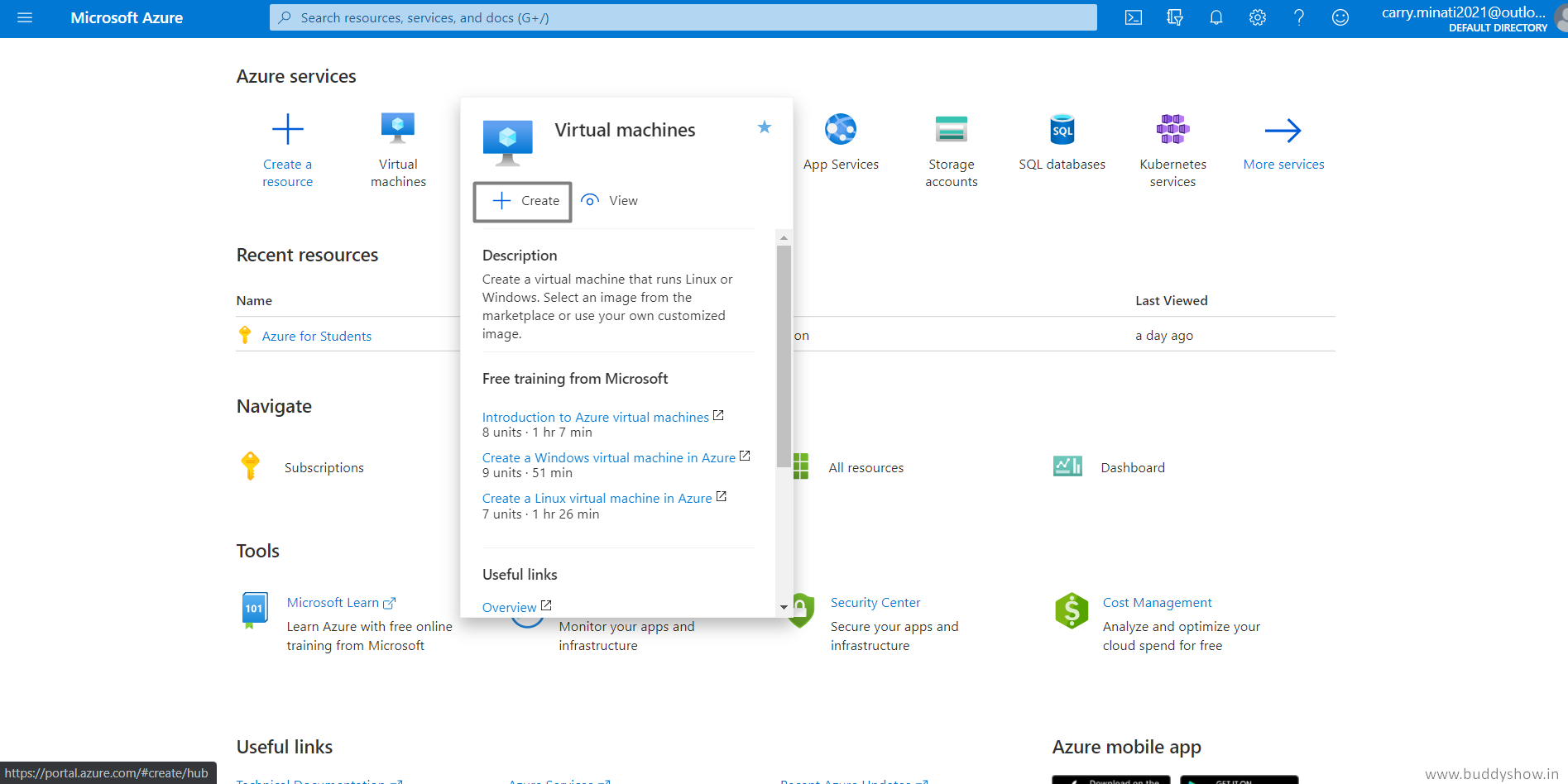The image depicts a comprehensive dashboard interface of Microsoft's Azure cloud platform. The top menu bar features a hamburger menu, a magnifying glass icon with the prompt "Search resources, services, and docs," along with a series of icons including a command prompt button, a bell for notifications, a gear for settings, a question mark for help, and a smiley feedback icon.

Highlighted elements in the dashboard include:
- A 2021 label next to "carry.menu" and "outlook."
- The "default directory" with options to observe services or create a new resource.
- A list of essential actions such as "Create a resource" and manage "Virtual machines."
- A resource named "Observe for Students."

Navigation tabs provide access to subscriptions, tools, and learning resources from Microsoft. These include "Microsoft Learn" and "Learn and Succeed," offering free online training and tutorials.

Specific courses listed are:
- "Introduction to Azure Virtual Machines" (8 units, 1 hour, 7 minutes)
- "Create a Windows Virtual Machine in Azure" (9 units, 15 minutes)
- "Create a Linux Virtual Machine in Azure" (7 units, 1 hour, 26 minutes)

Prominent sections of the interface are color-coded in blue, featuring categories like "App services," "Storage account," "SQL databases," and "Kubernetes services."

Additional functionalities provided include cloud resources, dashboard views, Microsoft security settings, cost management, and useful links. An Azure mobile app option is also visible, further enhancing accessibility and user experience.